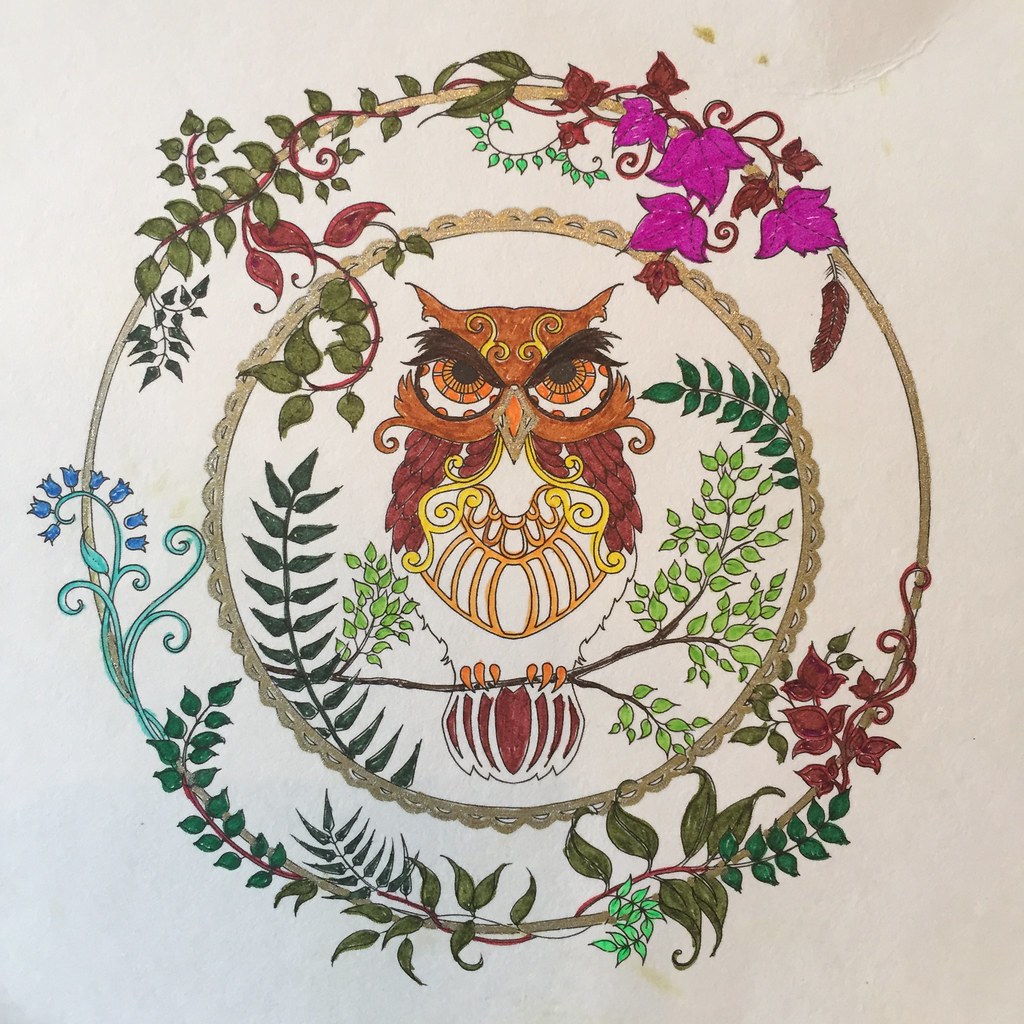This vibrant color illustration features a prominent owl at its center, immediately capturing attention with its strikingly large orange eyes and distinctive bushy, feathered tufts above them that resemble eyebrows. The owl's plumage is rendered in rich shades of brown, accentuated with intricate yellow and orange geometric patterns, giving it a unique and stylized appearance. Perched gracefully on a brown tree branch adorned with lush green leaves, the owl exudes a sense of watchful tranquility.

Surrounding the owl is an ornate, lacy circle that adds a delicate, intricate frame to the central figure. Beyond this, an outer circle is elaborately decorated with a variety of leaves and flowers, showcasing a vibrant palette of reds, purples, and blues. These elements combine to create a harmonious and aesthetically pleasing border that enhances the overall composition.

The artwork is presented on a piece of white paper, lending a clean and classic background to the illustration. However, the paper shows subtle signs of handling, including some fold marks and wrinkles near the top right corner, adding a touch of character and indicating that it is a well-loved piece. The image contains no text, allowing the detailed and colorful visual elements to speak for themselves.